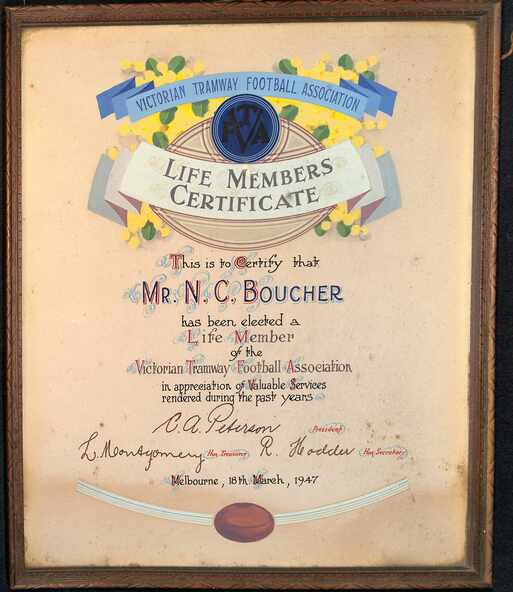This is a framed Victorian Tramway Football Association Life Member Certificate from March 18th, 1947. The certificate itself is displayed on a yellowing beige paper, which appears distressed with age. At the top, there is a prominent blue banner featuring the association's name and its blue oval logo with the black letters "FTVA". Enhancing the design, there is an array of yellow flowers with green leaves. Below the blue banner, an additional white banner announces "Life Member Certificate". The main body of text certifies that Mr. N.C. Boettcher has been elected a life member of the association in recognition of valuable services rendered. The text is in black, complemented by red embellishments. At the bottom, there are several signatures, including C.A. Peterson (President), L. Montgomery (Treasurer), and R. Hodeer (Secretary), followed by the date "Melbourne, 18th March 1947". Additionally, beneath the signatures, there is a distinct football shape in brown with a white curve marking. This significant recognition is encased in an elegant brown wooden frame.